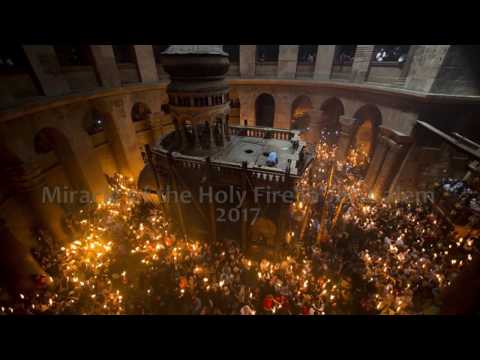The image captures the "Miracle of the Holy Fire in Jerusalem, 2017," prominently noted in a very light gray watermark at the top center. The scene is set at nighttime inside what seems to be an ancient stone structure, possibly resembling a stadium or a large ecclesiastical space. This structure, viewed from an aerial perspective, is characterized by wrapping medieval columns and arches around its periphery, which cast dark shadows under the night sky. 

In the very center of this vast, historic edifice, a raised stone platform with a tower-like architecture, reminiscent of designs seen in the Lord of the Rings, stands prominently with an opening at the top. Below this central stone structure, there is a large crowd of people gathered closely together, holding what appear to be torches or candles. These numerous light sources create a vibrant, illuminated sea of lights at the ground level. The flames vary in color from yellow to orange, particularly more pronounced on the left side, casting an orangish glow on the surrounding stone architecture. The people are barely visible amidst the lights, emphasizing the overwhelming luminosity in the image against the dark backdrop.